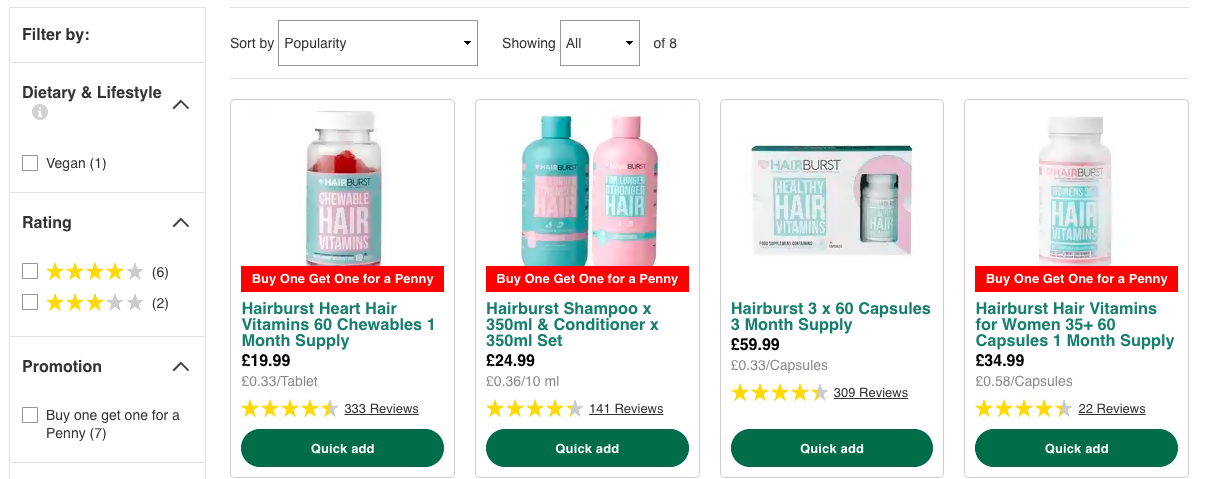The image is a screenshot of an online store's product page. The left sidebar features various filters: "Filter by Dietary & Lifestyle" with a single option, "Vegan," followed by "Filter by Rating," showing six products with four-star ratings and two with three-star ratings. Below these, a promotion filter "Buy One Get One for a Penny" lists seven qualifying items. 

The product display is sorted by popularity and shows eight items, with four visible at the moment and four more not currently shown. 

The first visible product on the left is prominently marked with a red text promotion, "Buy One Get One for a Penny." This product is a bottle of "Hairburst Heart Hair Vitamins" containing 60 chewables for a one-month supply, priced at £19.99. It boasts a rating of 4.5 stars from 333 reviews. A green "Quick Add" button is placed beneath it.

To the right is another highlighted product, a teal and pink bottle set. This set includes "Hairburst Shampoo X 350 milliliters and Conditioner X 350 milliliters," priced at £24.99.

The overall design and layout of the page emphasize ease of navigation and promotion highlights, aiming to attract health-conscious consumers seeking hair care products.